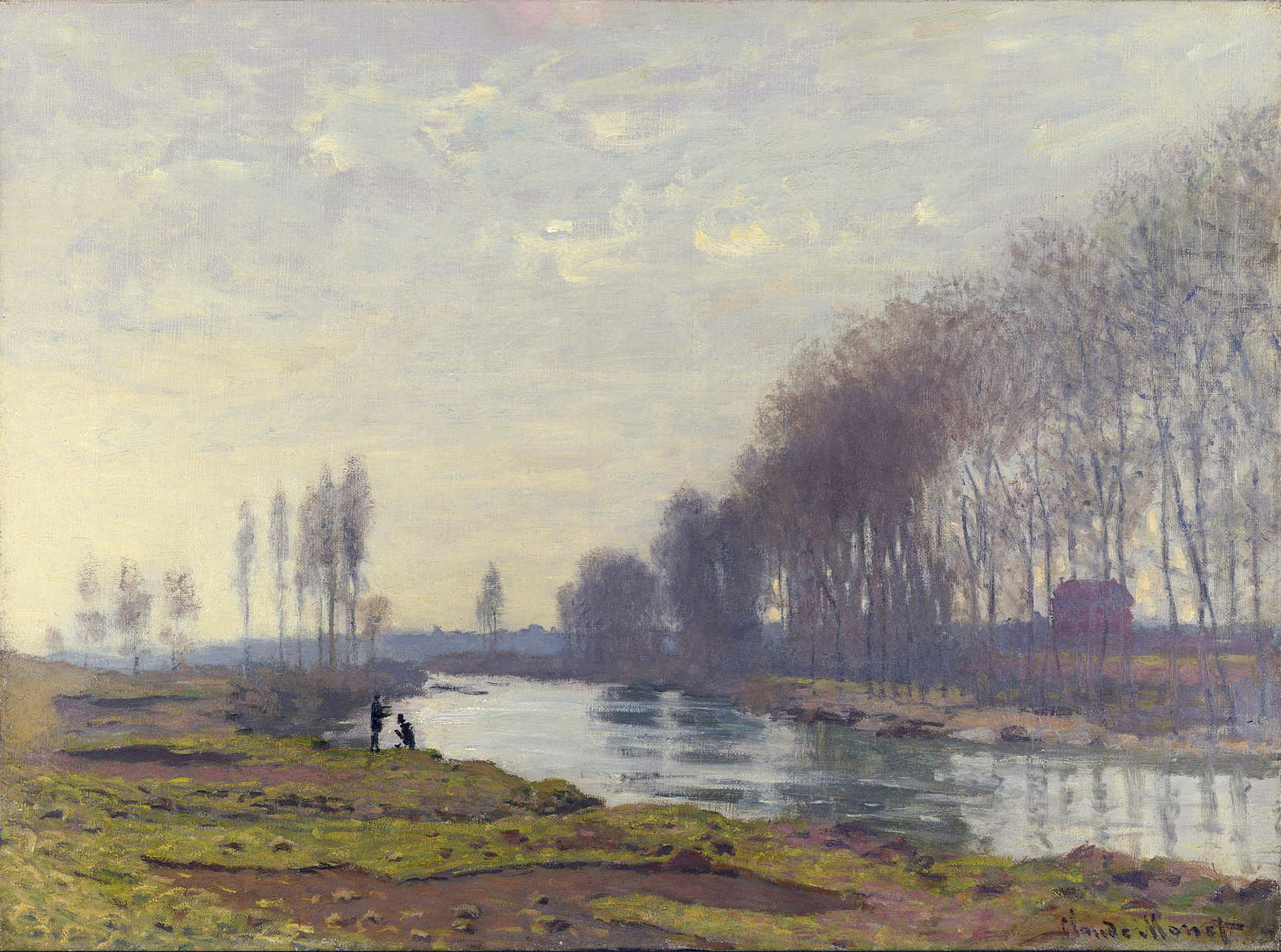This impressionistic painting, reminiscent of Monet's style, depicts a serene landscape featuring a light blue and white river extending from the bottom right towards the center. The sky above is moody with blues, whites, and hints of stormy clouds. On the left side, a grassy bank with uneven light green grass and patches of dark brown dirt stretches along the river's edge. The right side of the scene is framed by a sparse tree line of very tall, thin wooden trees with faint green and brown leaves near their tops. In the distant background behind these trees, a red building subtly peeks through. In the bottom left corner, two small black silhouettes can be seen by the riverbank—one figure kneeling and facing left, and the other standing and facing right, possibly engaged in a quiet activity like fishing. The painting beautifully captures the essence of perspective and tranquility in an idyllic natural setting.